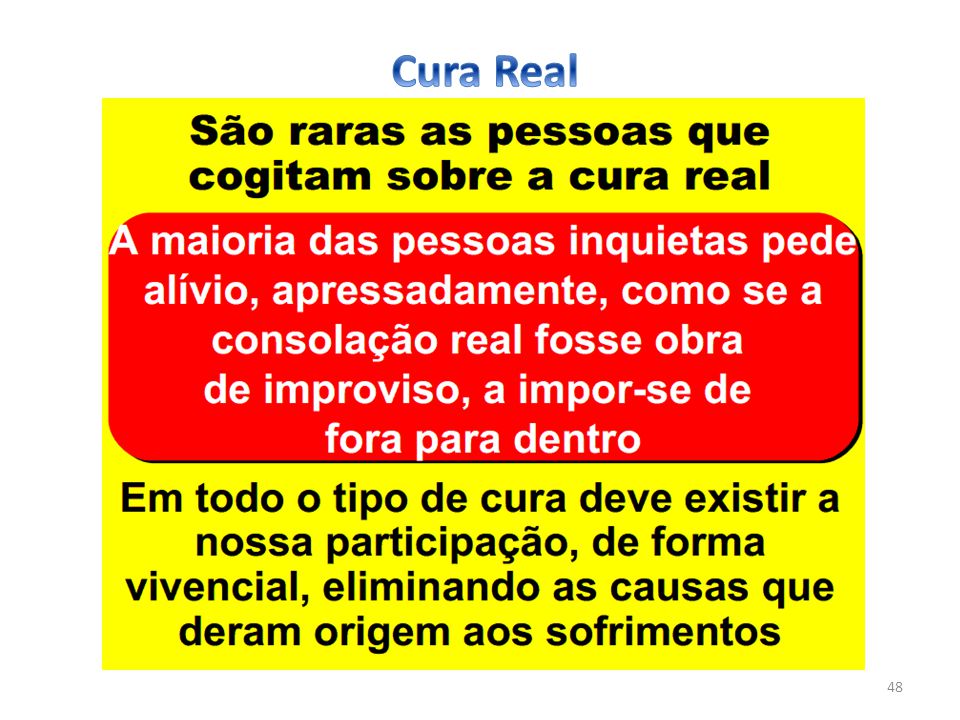The image appears to be a stylized text-heavy design reminiscent of a PowerPoint slide, with various sections distinguished by background color and text formatting. At the very top of the image, there is a prominent blue text that reads "CURA REAL" (C-U-R-A space R-E-A-L). Below this, on a yellow background, is a section containing heavy and thick black text that is difficult to read, presumably in Spanish. The middle section of the slide has a red background with white text which features phrases like "INQUIETA SEDE ALIVIO A PRESSADAMENTE" and "Como se a CONSOLAÇÃO Real Fosa Obra de IMPROVISO a imporse de forma para dentro." The bottom section of the slide returns to a yellow background with thinner black text, continuing in the same language. The font changes in thickness from the top to the bottom of the image, with the heaviest font at the top and progressively lighter fonts towards the bottom.